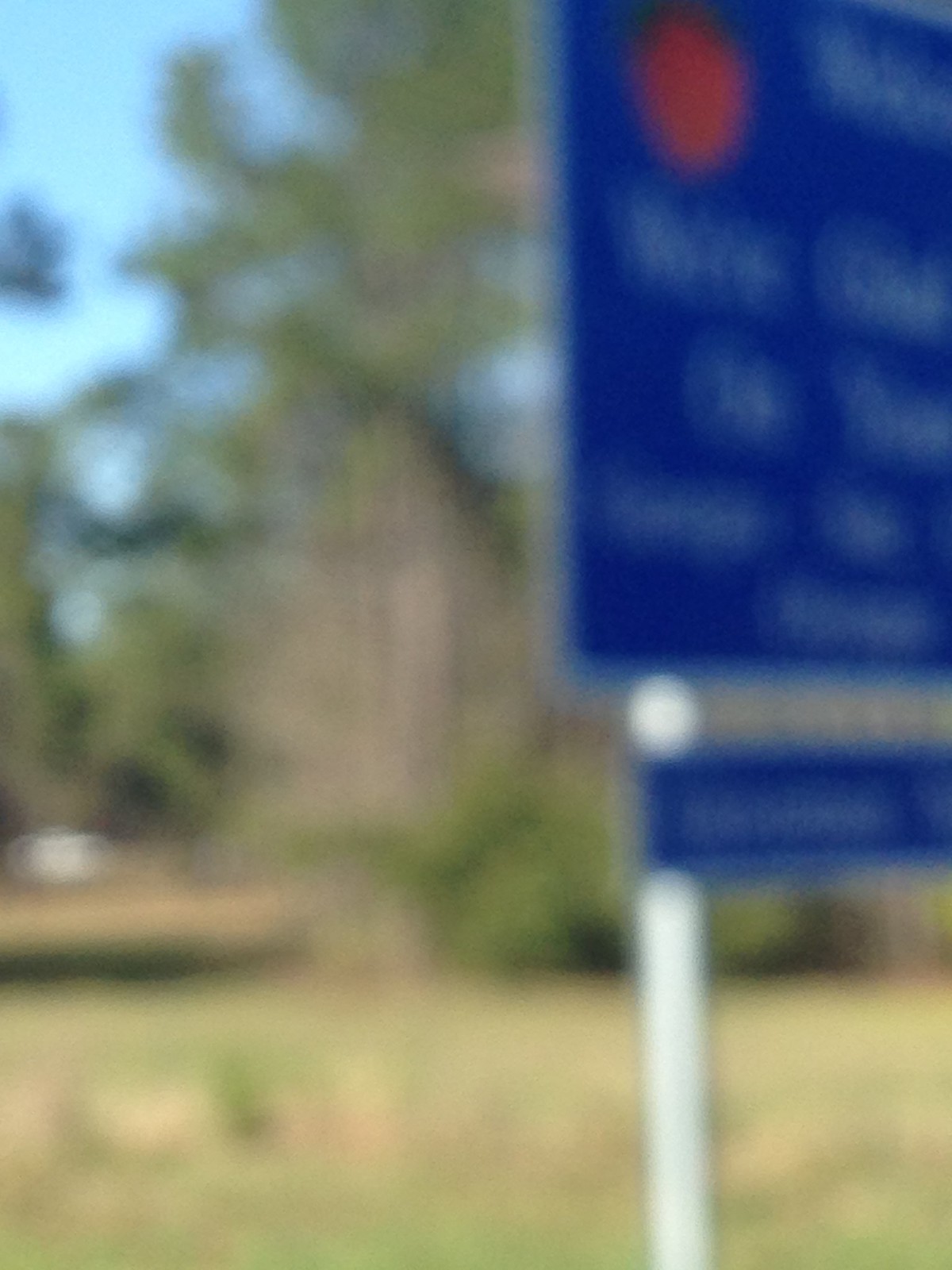This image portrays a blurry rectangular photograph taken outdoors in portrait orientation. Central to the image is a blue road sign mounted on white poles, partially cut off on the right side. The sign appears to consist of two sections: a larger main portion with a white border and illegible white writing, and a smaller, narrower section beneath it. Both sections perhaps delineate the location as a park or rest area. Notably, there is a distinct, bright red dot on the sign, although any text or further details remain unreadable due to the poor focus.

The backdrop features a grassy area with some parts appearing brown, possibly indicating a summer setting. In addition to grass, there are various green bushes and a couple of tall trees with green foliage extending into a clear blue sky, suggesting daytime conditions. On the left side of the image, there is an indistinct white object that might be a parked car or another element in the scene.